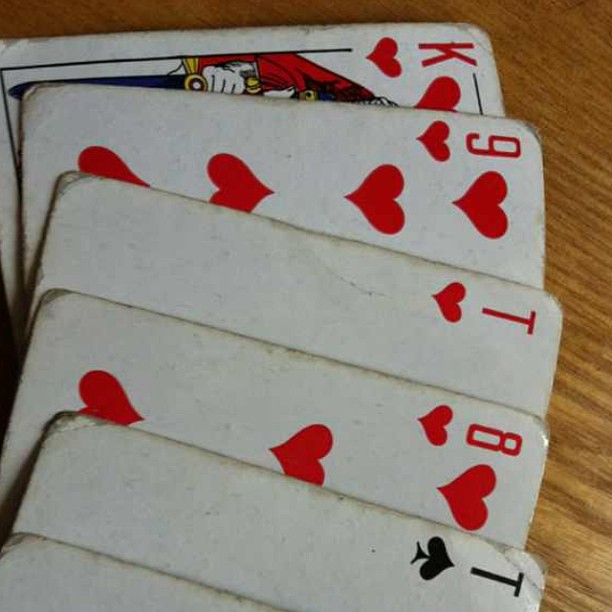A timeworn deck of six playing cards lies scattered on a rustic wooden table, their age and frequent use evident from the rounded, frayed corners and various stains. Although the value of the bottom card is obscured, the card above it is clearly the Ten of Spades, distinguishable by a large, black “T” with an extended stem and a spade symbol beneath it. Next to the Ten of Spades is the Eight of Hearts, featuring a red “8” and a heart symbol in the upper left corner, accompanied by three hearts on its face—two upright, one inverted. Beside it is the Ten of Hearts, identifiable by its similarly designed “T” and heart symbol. Above the Ten of Hearts lies the Nine of Hearts, showing a red “9” and heart symbol along with four visible hearts—two upright, one inverted. The topmost card offers a tantalizing glimpse of the King of Hearts, with a large “K” and a heart symbol, plus a portion of the illustration depicting the king gripping a sword.